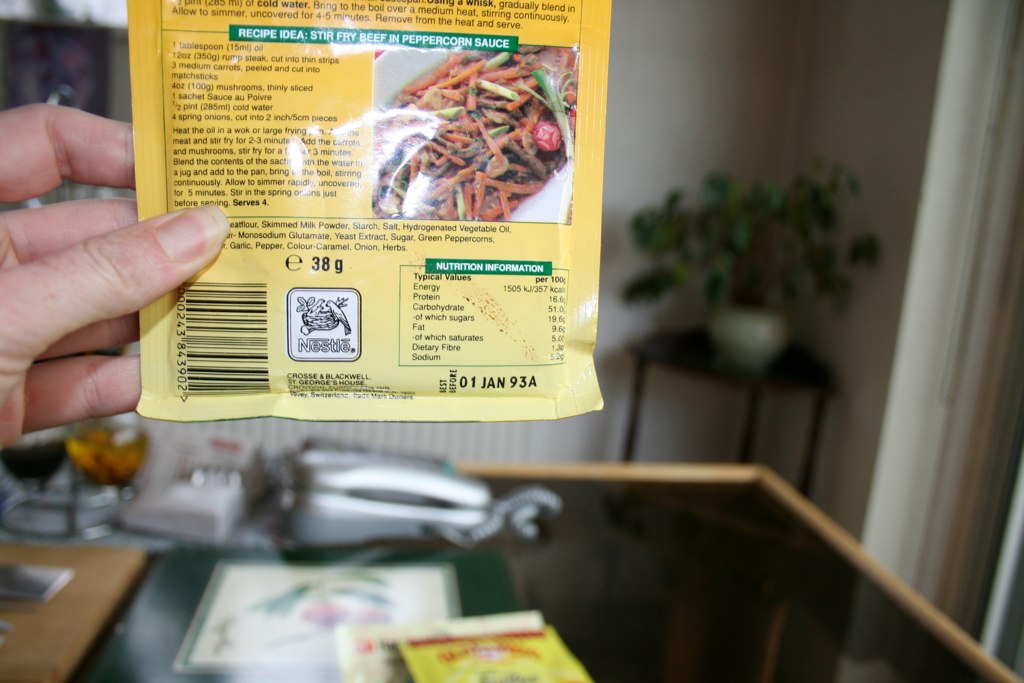The image shows a person with white skin tone and long fingernails on their thumb holding a yellowish, squarish seasoning packet made by Nestle, which weighs 38 grams. The packet features a recipe idea for stir-frying beef in peppercorn sauce, alongside other items like carrots, and has an expiration date of January 1, 1993, indicating its age. The scene is set indoors in a brightly lit home, suggesting it is daytime. In the background, there is a green potted plant and at the bottom middle of the image, a glass coffee table with several objects on it, including a silver phone.